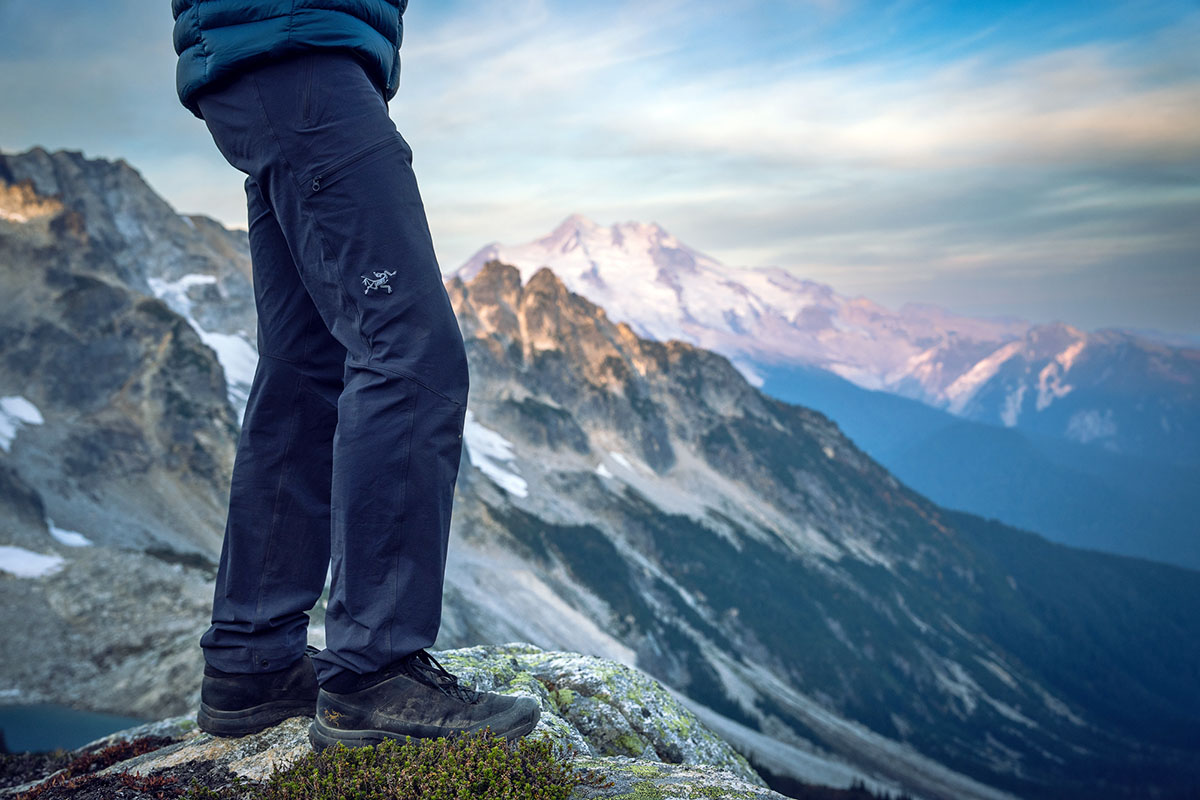This photograph showcases a hiker standing on a weathered, rocky outcrop overlooking a stunning mountain range. Captured from the waist down, the hiker is attired in a dark teal puffy jacket, only the bottom of which is visible, paired with navy blue hiking pants that feature a light blue logo above the knee and a zipper pocket on the right leg. The hiker's black, low-topped hiking shoes, worn and dust-covered, rest on the gray rock dotted with patches of green moss and lichen.

In the midground, the rugged mountains extend from the upper left to the lower right, showcasing their dramatic, snow-streaked peaks with hints of yellow sunlight gracing one in the middle. Further in the distance, an additional ridge of entirely snow-covered mountains adds depth to the landscape.

The vibrant blue sky, adorned with wispy cirrus clouds, forms a picturesque backdrop, highlighting the vast, snow-covered terrain and emphasizing the altitude and solitude of the location. This detailed portrayal conveys the serene yet majestic beauty of a high-altitude adventure.